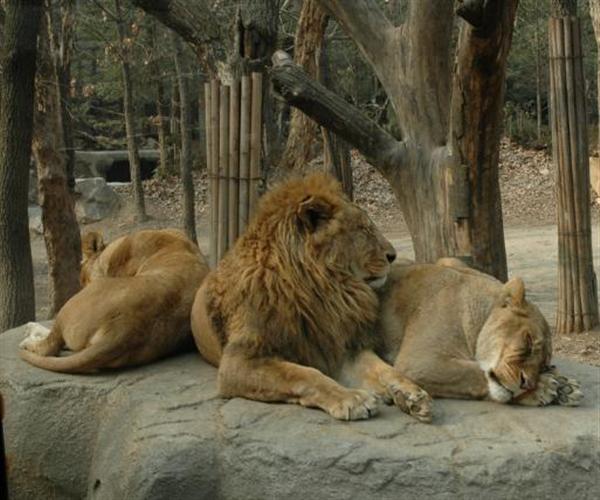This image is a color photograph in landscape orientation, capturing three lions resting on a large, flat, grayish rock within a zoo enclosure. The central figure is a male lion with a short brown mane and a beige coat. He is reclining with his front paws stretched out toward the viewer and his eyes closed, looking peaceful as he faces the right side of the image in profile. To the male lion's right, a female lioness is sleeping, her head resting on her paws near the right edge of the image. On the left side, another female lion is also laying down, with her back to the viewer and her tail curled around near her paws. The background of the photograph features several tied bamboo poles and various tree structures, adding an intentional and structured feel to the lion's habitat. The overall atmosphere exudes tranquility and natural realism, depicting the serene rest of the three lions within their meticulously arranged zoo environment.